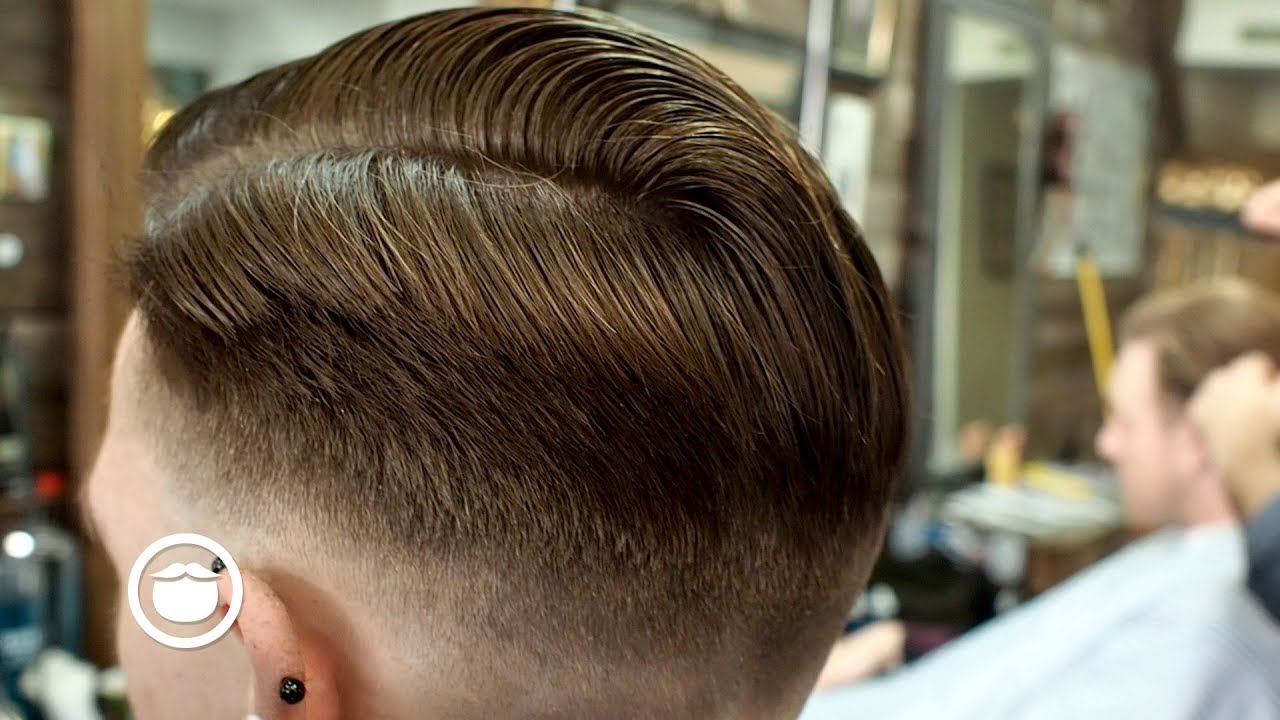The photograph showcases the inside of a barbershop, focusing primarily on the head of an individual who has just received a haircut. The person's head fills the left two-thirds of the image, and they have a conservative short haircut with visibly more hair on top and very short hair around the sides and back. The hair is brown with a tint of red, parted from the right to the left. The left ear of the person is prominently featured, displaying two small black circular piercings—one on the side and one on the top of the ear.

In the blurred background on the right side of the photo, another individual is visible, also receiving a haircut. We can see the hands of the barber working on their hair, and they are covered with a classic white barbershop gown. Behind the person in focus, there are mirrors on the wall that reflect parts of the scene. In the lower left corner of the image, there is a distinctive logo: a round white circle containing the image of a beard and mustache, reminiscent of the traditional Santa Claus look, which appears to be the emblem of the barbershop.